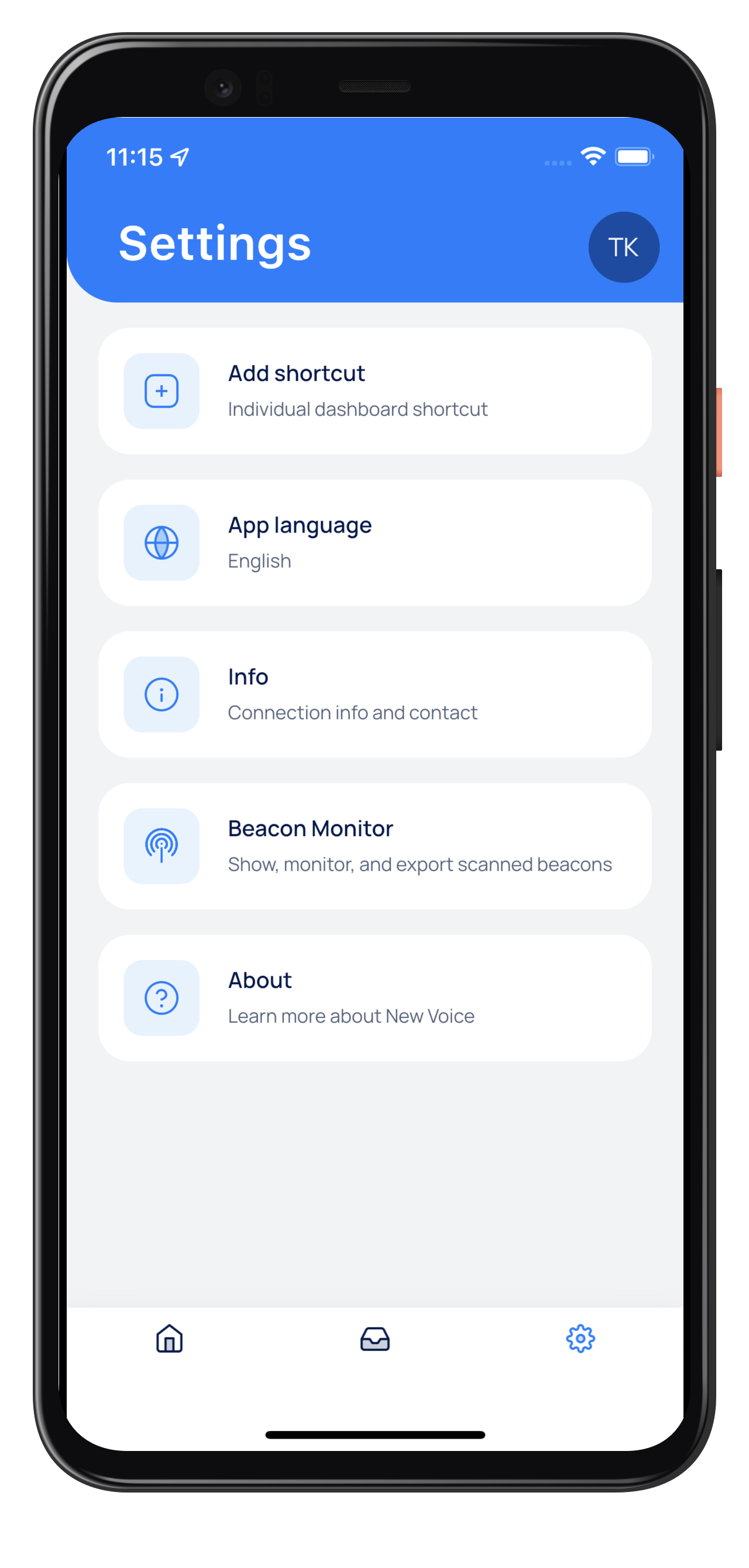The image depicts the settings menu on what appears to be an older model iPhone, characterized by its black candy bar design and relatively thick bezel. The screen shows a detailed settings interface, with the top 15-20% of the phone's outline clearly visible on the display.

At the very top, the status bar is set against a blue background with white text, showing the time as "11:15" alongside the location icon, four dots indicating cellular signal strength, a fully lit Wi-Fi signal, and a full battery indicator.

Just below the status bar, aligned to the left in white text, is the heading "Settings." Adjacent to this, on the right side, is a dark blue circle containing the white letters "TK."

The main section of the screen lists five different settings options against a white background:
1. **Add shortcut** - Includes an icon with a plus sign inside a box to the left.
2. **Individual Dashboard Shortcut** - Also with a plus sign icon in a box on the left.
3. **App Language: English** - Featuring a globe icon to the left.
4. **Info Connection and Contact** - With an information symbol to the left.
5. **Beacon Monitor** - Described with "Show, monitor, and export scanned beacons," accompanied by a beacon icon to the left.
6. **About** - Noted as "Learn more about New Voice," with a question mark icon to the left.

At the bottom of the screen, there are three navigation icons for Home, Download, and Settings. The Settings icon is highlighted in blue, while the Home and Download icons are in black.